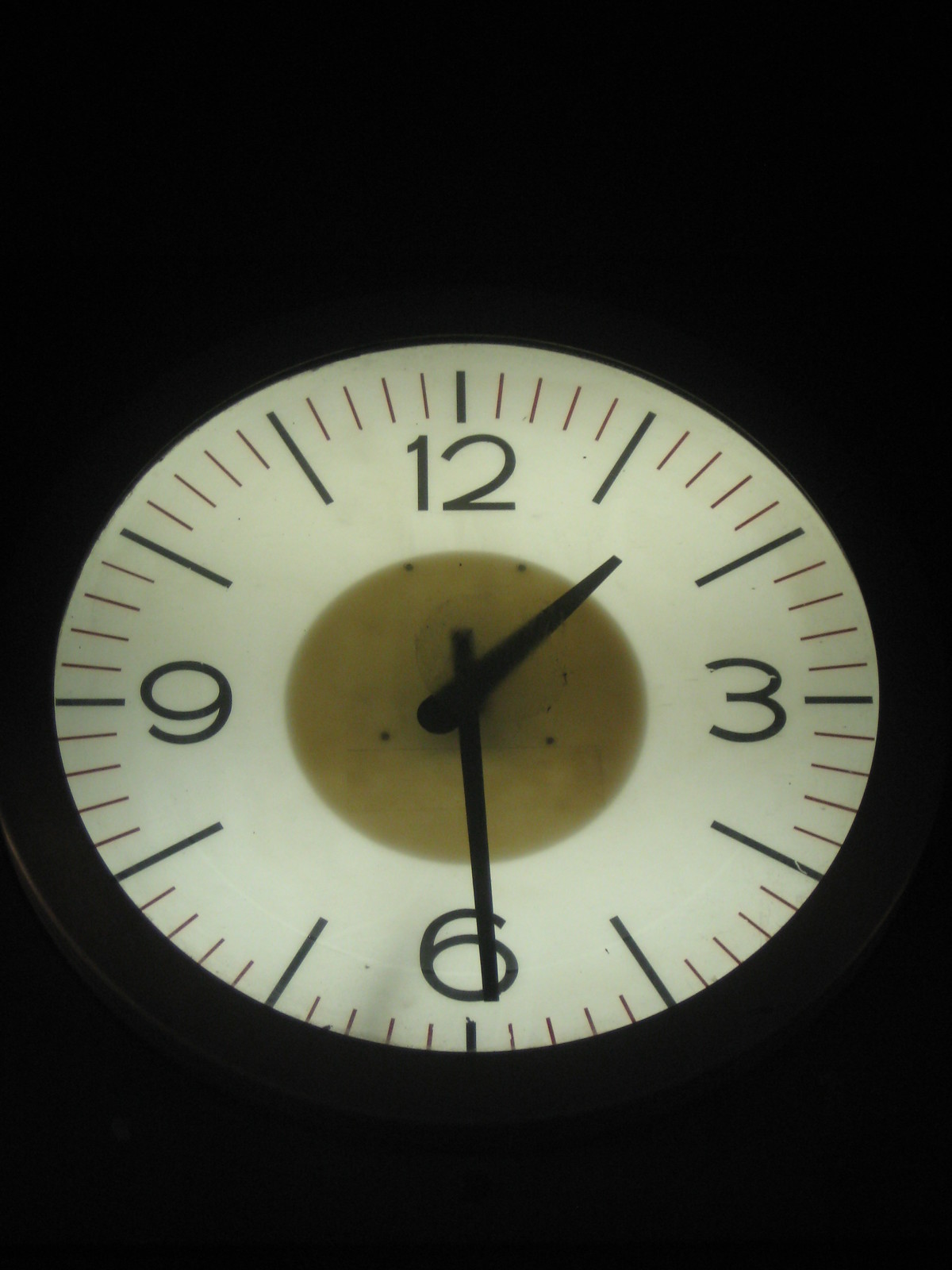The image displays a round clock against a completely black background, which might be a black table or simply an effect of the photograph. The clock features a thin black frame around its white face. The hour markers and the large numbers at 12, 3, 6, and 9 are in bold black, while the minute markers, appearing at five-second intervals, are small red lines. The current time displayed is approximately 1:28. At the center of the clock, there's a smaller circle in a distinctive greenish-yellowish-brownish hue, resembling a pea soup color. The clock hands for the hour and minute are also black, clearly standing out against the white background.